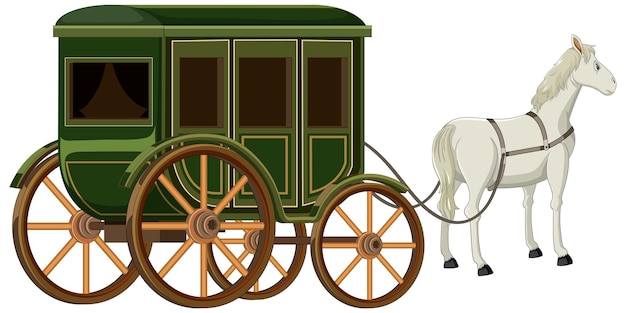This image, designed in a cartoon style with a white background, features a white horse with a rounded face and black hooves, facing right. The horse has a strap or reins around its head and body, attached to a classic, enclosed 18th-century-style carriage. This green carriage, depicted with four wooden wheels—brown in color with slightly peach-colored spokes and centers—shows a slight inconsistency in size as the back wheels are larger than the front. The carriage itself is dark green with lighter green highlights and brown windows, adorned with curtains inside. The detailed image captures the nostalgic design elements, including the brown and peach accents on the wheels, giving it a charming, slightly out-of-proportion quirkiness.